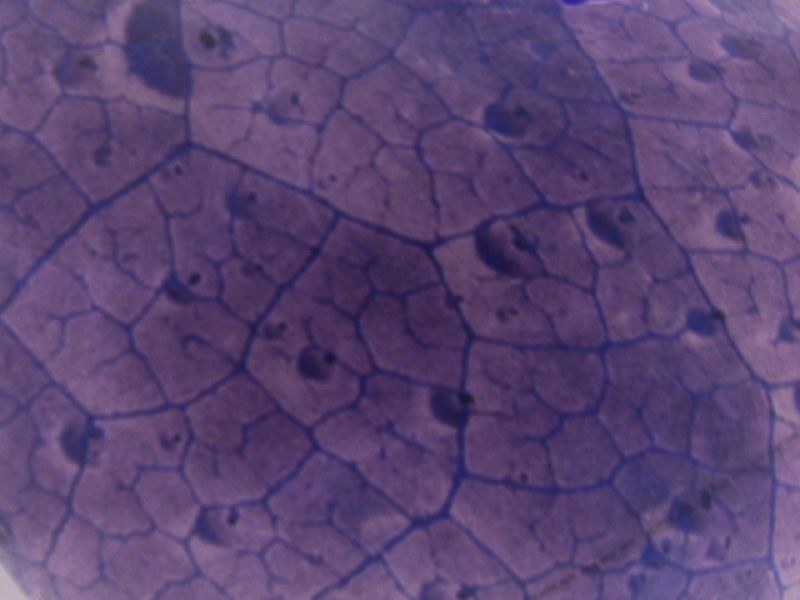The image is a rectangular close-up, predominantly purple, resembling the view through a microscope. The main features are numerous shapes—squares, rectangles, and octagons—bordered by dark blue lines with some bumpy and cracked textures. Dark purple spots and splotches are scattered throughout, contributing to an uneven, almost aged appearance. The overall effect is reminiscent of the structure of dry skin cells or brain tissue, with veins or cracks creating an intricate, vein-like pattern. The purple shades differ in intensity, with the borders and interior shapes contrasting sharply, making the surface look textured and complex.